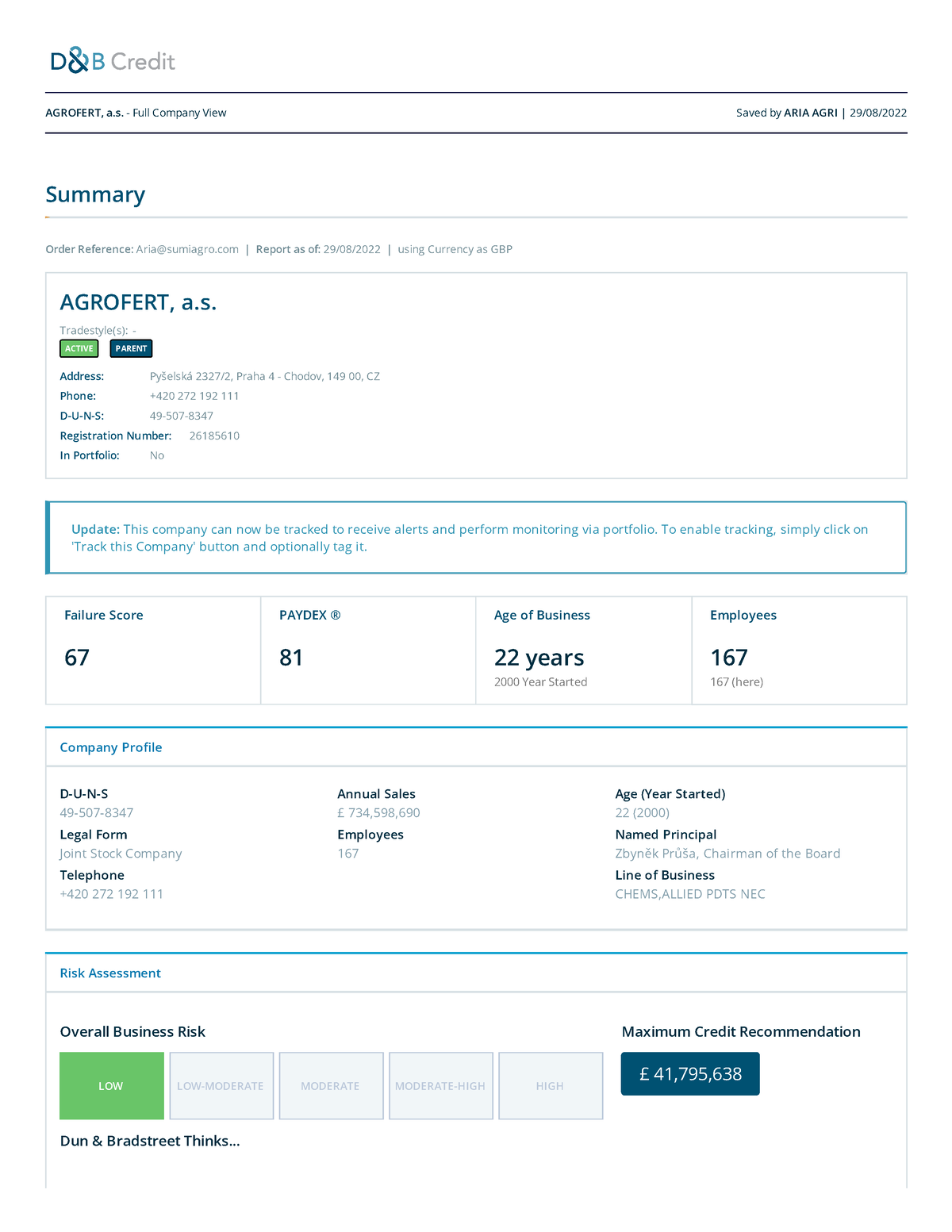This screenshot depicts a webpage from D&B Credit, distinguished by its company logo in the upper left corner, featuring a unique two-tone blue design incorporating the letters 'D', '&', and 'B' in a distinctive pattern. Directly beneath the logo is a line of information, which appears to be too small to decipher, potentially providing a breakdown of current site users. The word 'Summary' is prominently displayed below in bold, bright blue font, making it highly visible. Accompanying this are smaller, illegible blue text entries. Dominating the middle of the page is a large rectangular section bordered by a gray line, which seems to present information about a specific company inquiring about its credit standings. The page seems to function as a credit rating summary, assisting businesses in evaluating their eligibility for a loan.